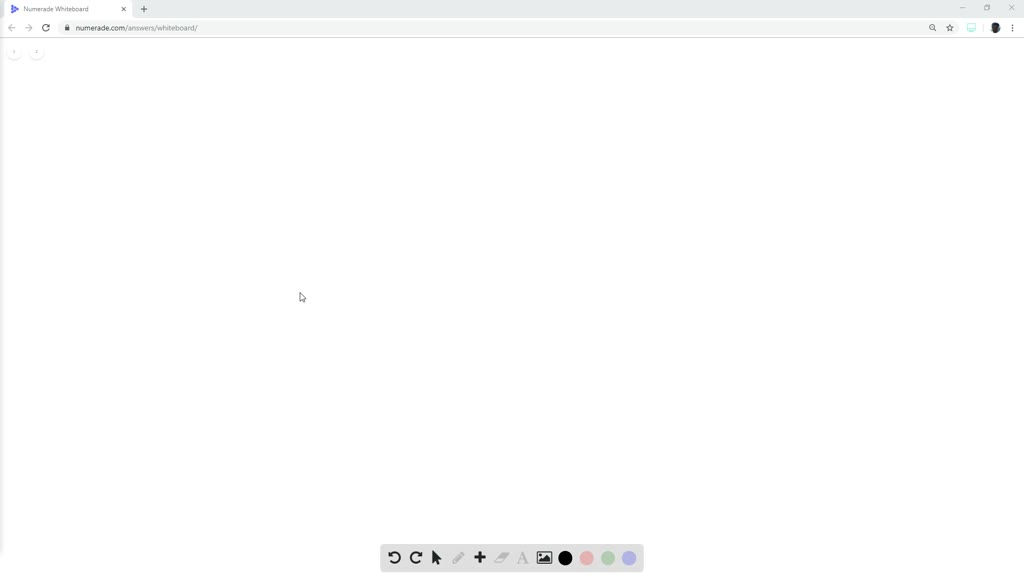This image is a detailed screenshot of a website. Prominently displayed at the top left of the screen is the URL bar, which shows the current address as "numeraid.com/answers/whiteboard/". Above the address bar, the browser tab label reads "Numerable Whiteboard", and it is distinguished as the only open tab.

Directly beneath the URL, there are two white, circular icons side by side; the first icon on the left contains the number "1", while the second icon on the right contains the number "2". The central area of the screen features a white mouse cursor hovering around the middle, indicative of user interaction.

At the bottom of the page is a gray, rectangular toolbar that contains various editing and drawing tools, consistent with a virtual whiteboard interface. This toolbar includes buttons for navigating backward and forward, selecting a mouse cursor, and inserting images. Additionally, it provides color options for drawing and writing, including black, red, green, and blue. The overall layout and features of the page suggest it is designed as a virtual whiteboard, likely intended for educational purposes, allowing users to draw, write, and make notes as one would on a physical whiteboard.